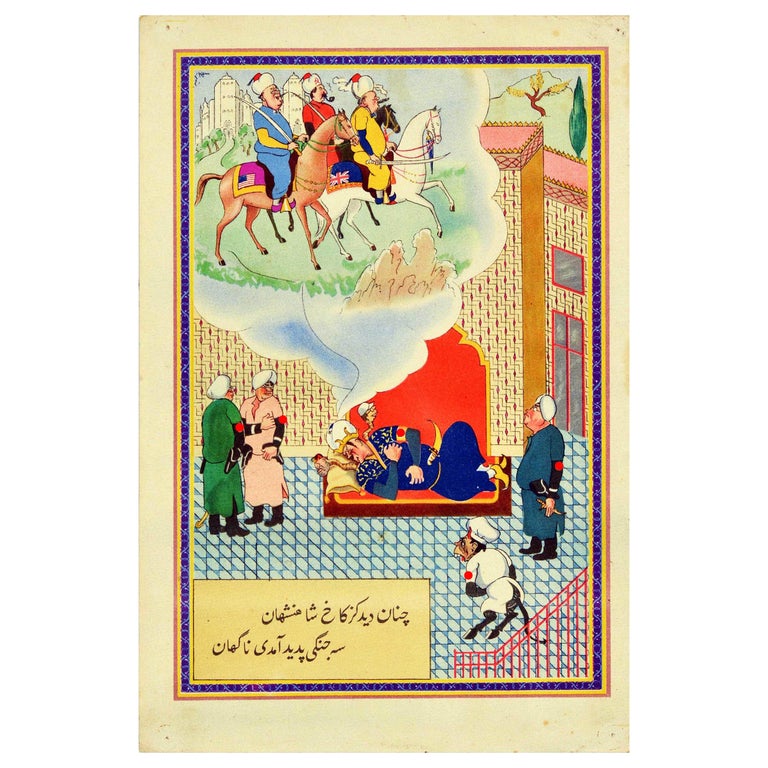The image is a detailed cartoon drawing set in a rectangular frame. At the center lies a man on a red-fabric-lined pallet or couch-bed, wearing a crown and a dark blue tunic adorned with a red circle symbol on his arm. He appears to be dreaming, with a thought bubble extending from his head that vividly depicts three men in traditional Middle Eastern or Ottoman attire, riding horses in front of a castle surrounded by trees. The first rider on a brown horse carries an American flag and sports a blue tunic with a yellow undershirt. The second rider, on a horse with a blue and red gold embroidered saddle, carries a British flag and wears a gold tunic with a dark blue undershirt. The third rider, partially obscured, has a red tunic with a dark undershirt. Each rider dons Arabic headgear with red tassels.

Two men stand to the left of the man on the pallet, one in a green tunic and the other in a pink tunic, both wearing traditional headgear and black shoes, with one carrying a golden scabbard. To the right, another man in a cyan dark blue tunic with a red arm symbol and similar headgear gazes at the thought bubble. Near the bottom right, an anthropomorphic, monkey-like creature dressed in a white tunic and a chef's hat observes the scene. Foreign script text appears in the bottom left, adding an exotic touch to the illustration.